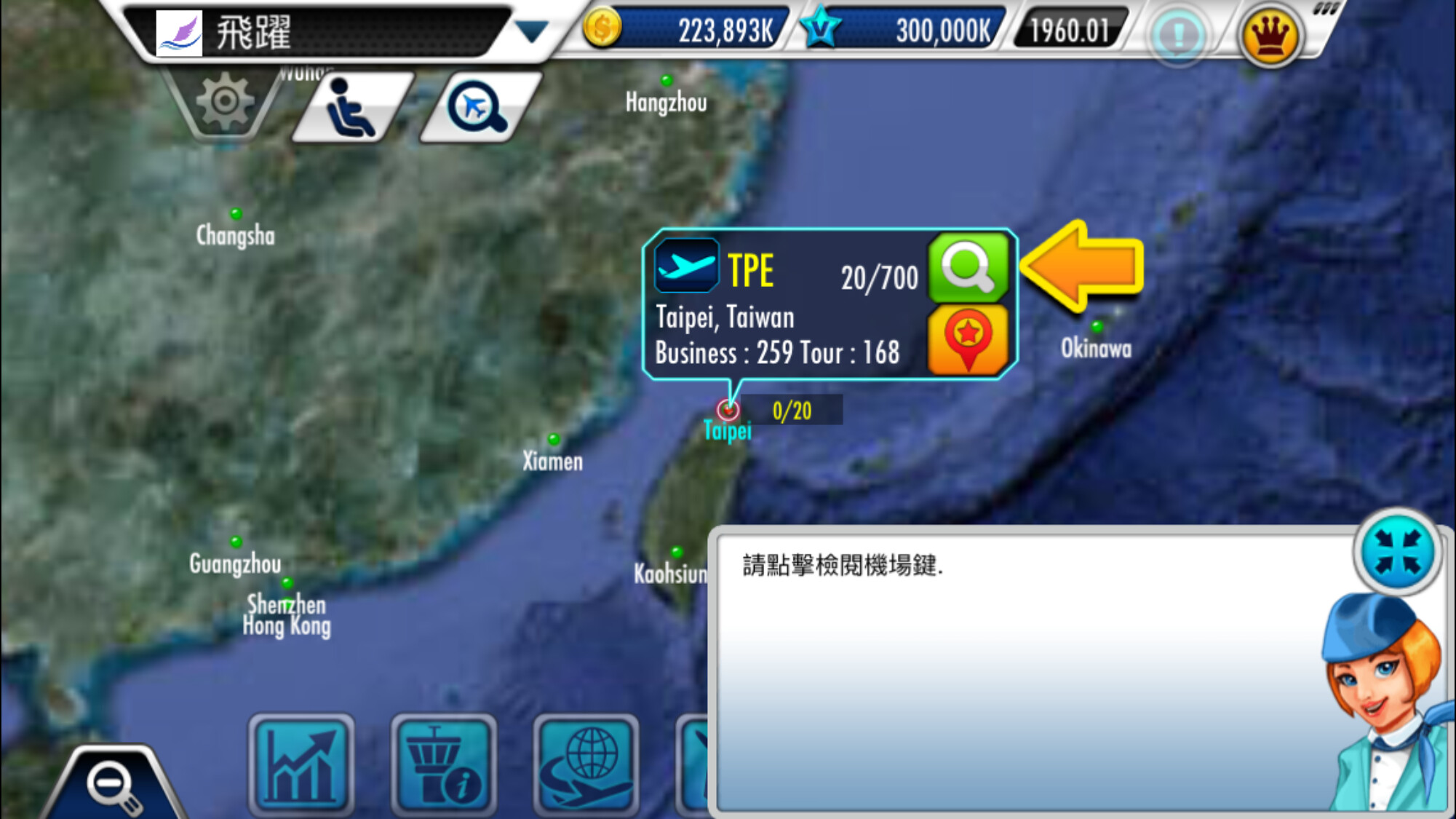The image is a detailed screenshot from a video game, likely set in a Chinese-speaking region, as evidenced by the Chinese characters in various parts of the interface. Dominating the background is a map that displays a landmass on the left and an oceanic area on the right. Prominent on the map is a rectangular box labeled "TPE Taipei, Taiwan" with additional details such as "Business 254 Tor 168 20-700," indicating possible travel options. An arrow points to Taipei, and the surrounding map shows other cities marked with dots and labeled in white, including Hong Kong. 

The upper left corner of the screen shows various in-game currencies, including $223,893 next to a gold coin, $300,000 next to a blue star, and $1,960.01. A blue airplane icon suggests navigational options for travel within the game. 

In the lower right corner, a character appears in a communication box. This character, presumably an AI-driven flight attendant, is depicted with short blond hair, blue eyes, and clothed in a blue coat over a white button-down shirt, complete with a blue cap. She seems to be engaging with the player, possibly offering information or assistance, indicated by the Chinese or Japanese text next to her image.